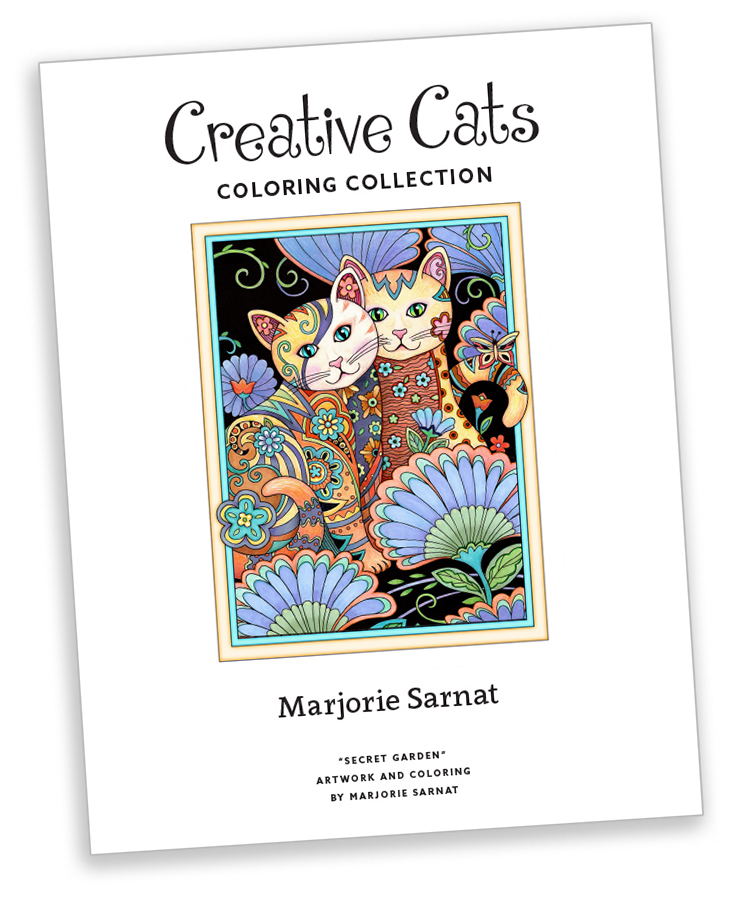The cover of this coloring book, titled "Creative Cats," features a whimsical black font at the top, reading "Creative Cats," followed by "Coloring Collection" in smaller, sans-serif black lettering. The background of the cover is solid white, focusing attention on the central, lavishly illustrated poster of two intricately designed cats. These cats, adorned in a variety of colors ranging from light tan to pink to deep brown, sit in a vibrant flower garden. The cat on the left is facing to the right with a tilted head and a smile, while the one on the right looks straight ahead. Surrounding them, blue and green flowers add an ornate touch to the already detailed scene. The author’s name, Marjorie Sarnat, is prominently displayed in black type beneath the illustration, with a smaller font below that reading "'Secret Garden' Artwork and Coloring by Marjorie Sarnat," showcasing her unique artistic style perfect for a coloring book.